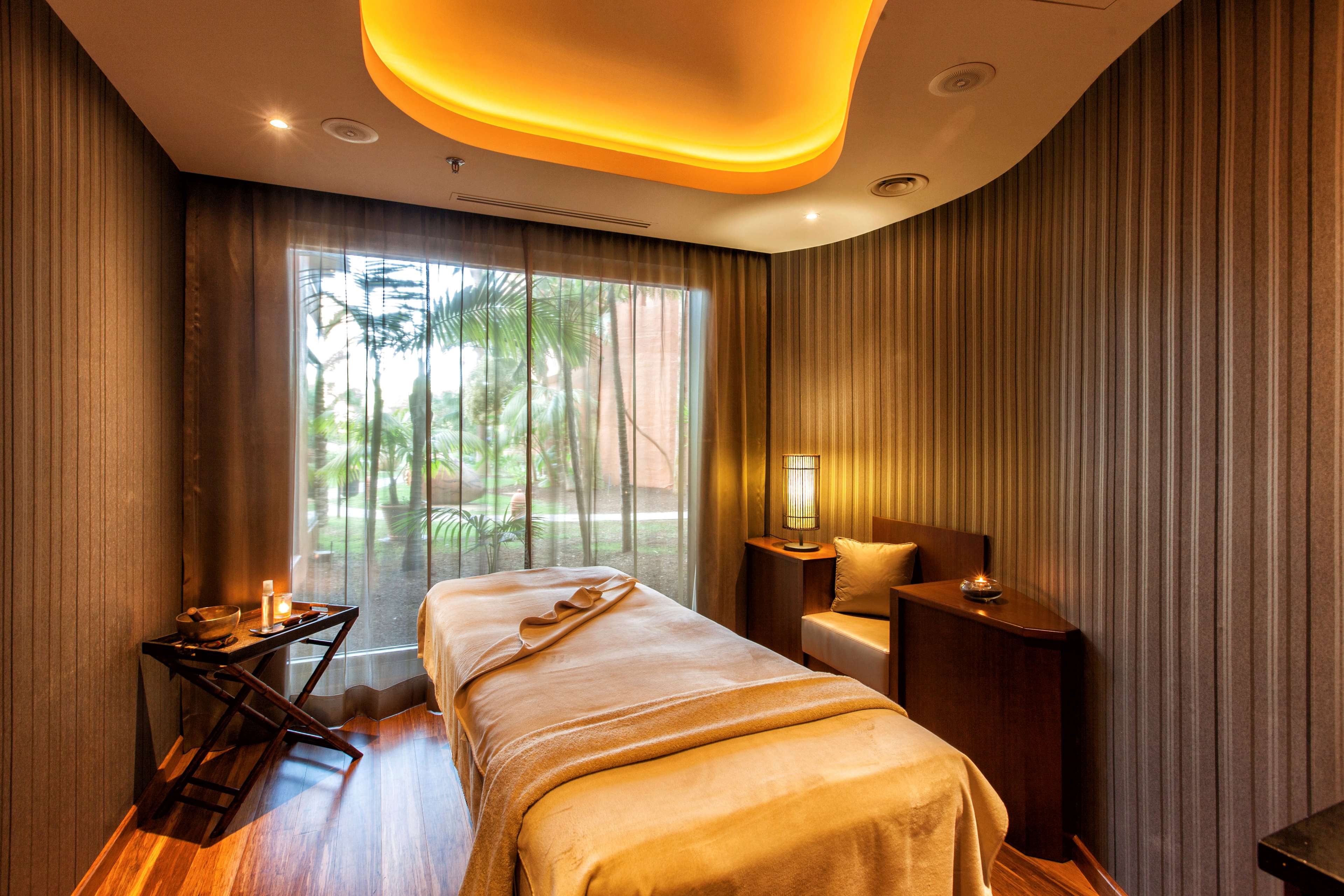This image depicts a serene, spa-like room, possibly located in a tropical setting, with elements suggesting both comfort and relaxation. The room features medium brown hardwood floors and walls adorned with vertical striped wallpaper in shades of white, gray, and black, creating a balanced and harmonious ambiance. Dominating the back wall is a large, balcony-style window covered with a sheer curtain, offering a picturesque view of an inviting courtyard filled with palm trees and other lush greenery. The sheer curtain subtly obscures the view of a nearby brick-colored building, adding to the room’s tranquil atmosphere.

In the center of the room is a twin-sized massage table, covered with a yellow sheet and topped with a folded, fitted orange sheet, indicating its primary function as a place for relaxation treatments. Adjacent to the seating area on the right, a built-in bench with a soft cushion is paired with a small side table holding a lit candle in a candle holder, enhancing the soothing environment. On the left-hand side, a folding tray table holds a golden bowl with a pestle, suggesting a setup for mixing massage oils or other spa treatments. Nearby, a small tray presents two oblong-shaped items resembling egg rolls, accompanied by a candle, possibly contributing to the spa's calming decor.

The amber-colored walls and a stylish ceiling light with rectangular form and curved corners, casting a warm yellow and orange glow, further enhance the relaxing atmosphere of the room. Overall, the blend of natural elements visible through the window, combined with the thoughtfully arranged spa accessories and furnishings, creates a harmonious and inviting space for unwinding and rejuvenation.